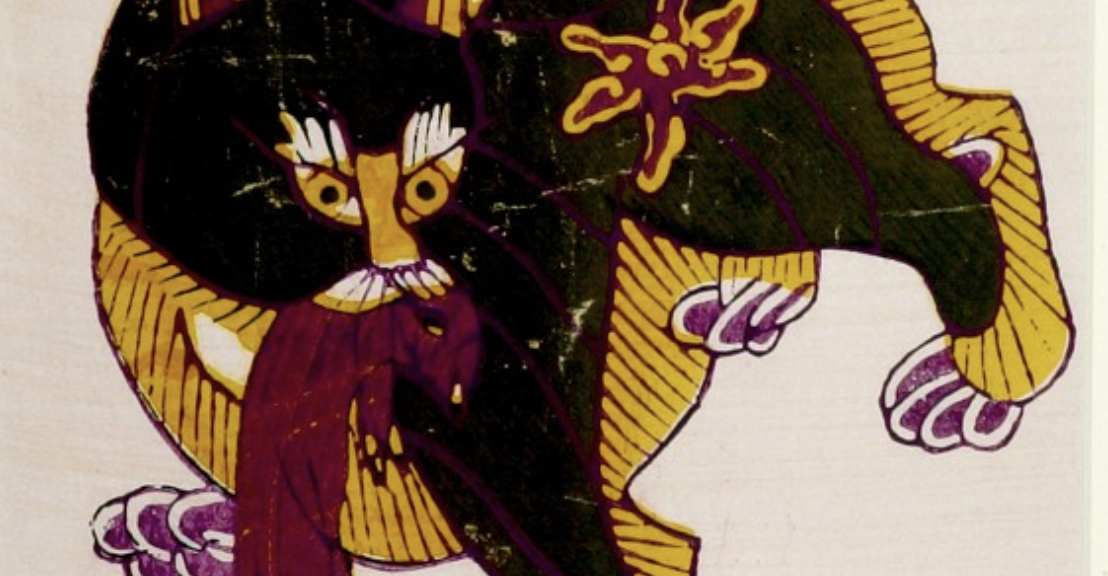This detailed artwork, likely created using markers or watercolors, depicts a cartoon-like creature resembling a feline, possibly a lion. The animal has a blend of black and yellow fur with maroon accents, including a distinct six-pointed star on its hind leg. It features large, golden-yellow eyes with spiky eyebrows in white and light yellow. The mouth appears to hold a purple-brown rodent-like figure, its body dangling downward. The creature's beard and mane are a bright pink and yellow. Notably, its paws are defined with white circles around each toe, adding an intricate purple detail. The image lacks any identifying information or context regarding the artist or its purpose. This enchanting piece is set against a cream or white backdrop, showcasing its vibrant colors vividly.